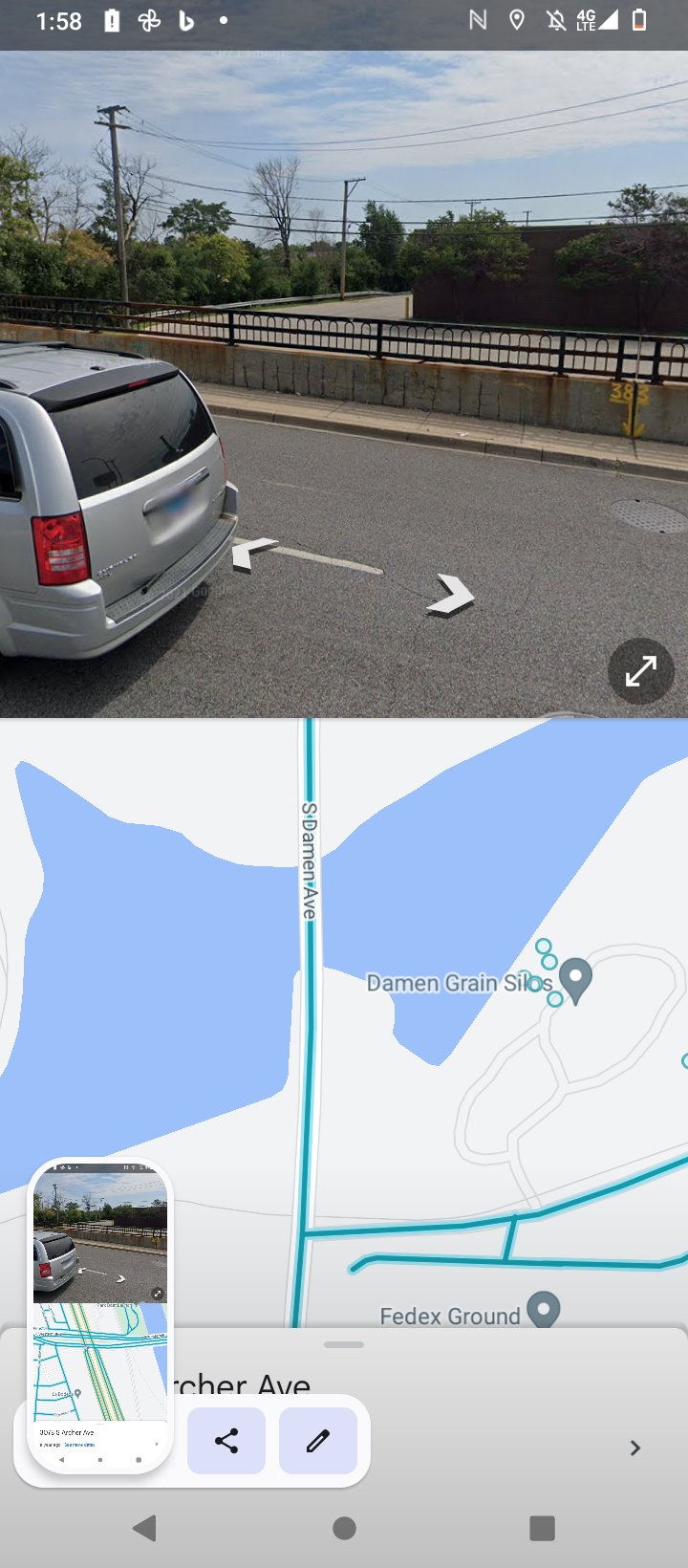The image captures a gray van in motion, taken on a smartphone as indicated by the visible top strip displaying the time, battery life, muted sound icon, and connection status. The van, characterized by its tinted rear windows and a blurred license plate, is traveling on a road marked with white directional arrows, suggesting turns available to the left and right. The background reveals a building partially surrounded by trees and adjacent to a parking lot, contributing to the urban scene. Complementing this snapshot, a secondary image on the phone displays a map with a route highlighted, identified as FedEx Ground, likely indicating the vehicle's delivery route or the tracker's journey monitoring their package.